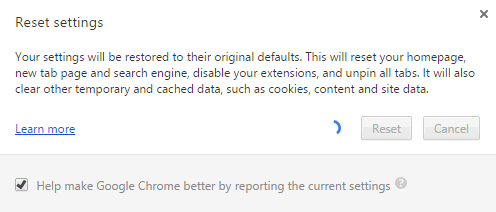The image appears to be a screenshot from a website, most likely Google Chrome. The background is predominantly white with dark grey text and a blue hyperlink. The text indicates an option to "Reset settings," and details that choosing this option will restore settings to their original defaults. This includes resetting the home page, new tab page, and search engine, disabling extensions, and unpinning all tabs. Additionally, it will clear temporary and cached data such as cookies and site data.

Beneath this explanation on the left side, there is another blue hyperlink labeled "Learn more." To the right of this link and to the left of the reset and cancel buttons, there is a partially visible blue circle, likely signifying a loading indicator, but only the right third of the circle is visible.

On the right side, there are two greyed-out buttons labeled "Reset" and "Cancel," indicating that they are currently not clickable. At the very bottom of the screen, there is a grey section with a checkbox option that reads "Help make Google Chrome better by reporting the current settings."

In the top right corner of the screen, there is an "X" icon to close out the page.